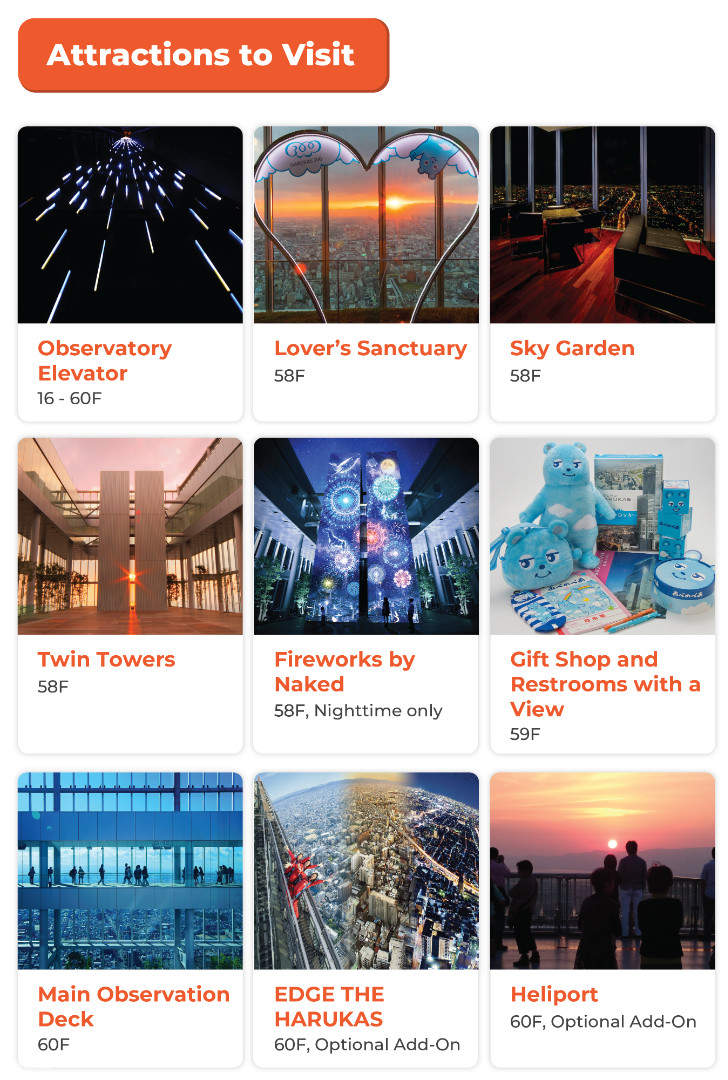The top right corner of the image prominently features the text "Attractions to Visit." The image details an observatory with an elevator that provides access from the 16th to the 60th floor. Highlighted on the 58th floor is the Lover's Sanctuary, marked by a heart-shaped archway. In the background, a beautiful sunset casts its glow over a cityscape brimming with numerous buildings. 

The Sky Garden, found on the 58th floor, is showcased with wooden elements accentuated in red hues. The iconic Twin Towers stand tall in the scene, with fireworks bursting in vibrant displays, visible only before nightfall. Adjacent to the main observation deck, visitors can explore walkways that edge the structure.

The image also includes glimpses of a gift shop and several restaurants that offer panoramic views. Blue bears and gray architectural details populate the background scenery. Furthermore, the hierarchy of floors includes an optional 64th-floor add-on, framed by a sky tinted with shades of red.